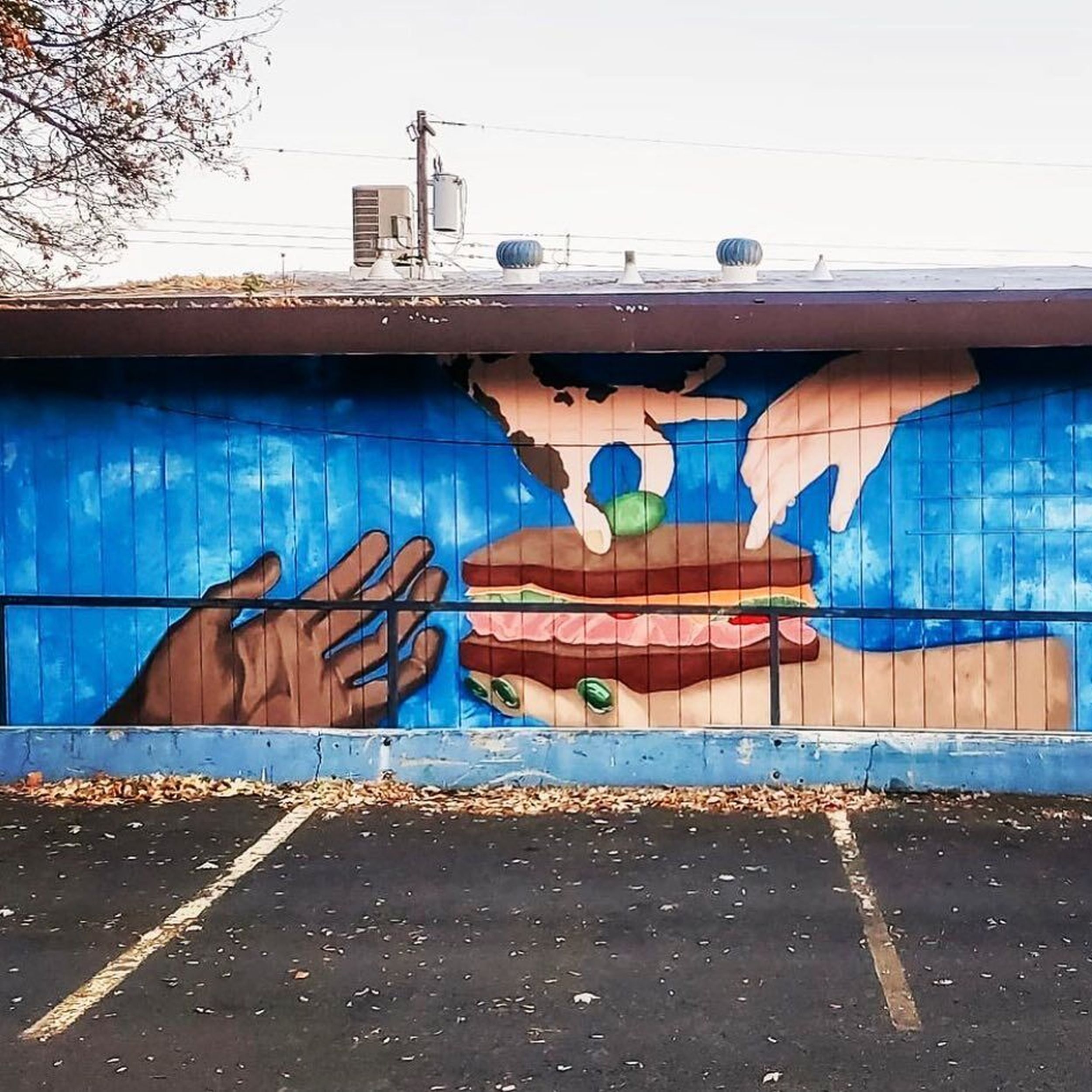This outdoor photograph captures a vividly detailed mural adorning the wall of an old building, behind a parking lot with clearly marked spaces and a metallic railing serving as a barrier. The building's slightly sloped roof is adorned with an AC unit, two circular vents, and is edged with dead leaves from an overhanging tree. The sky above appears white, and electrical poles and lines are visible in the background.

The mural itself features a striking blue backdrop and depicts four hands of various shades of brown. A hand from the bottom right holds a large sandwich, resembling a ham and cheese sandwich topped with an olive. Two hands above appear to delicately touch the top piece of bread, while a darker hand from the bottom left extends towards the sandwich, as if reaching out for it. Each hand is painted with care, showcasing the different hues and uniting them in the act of sharing the meal.